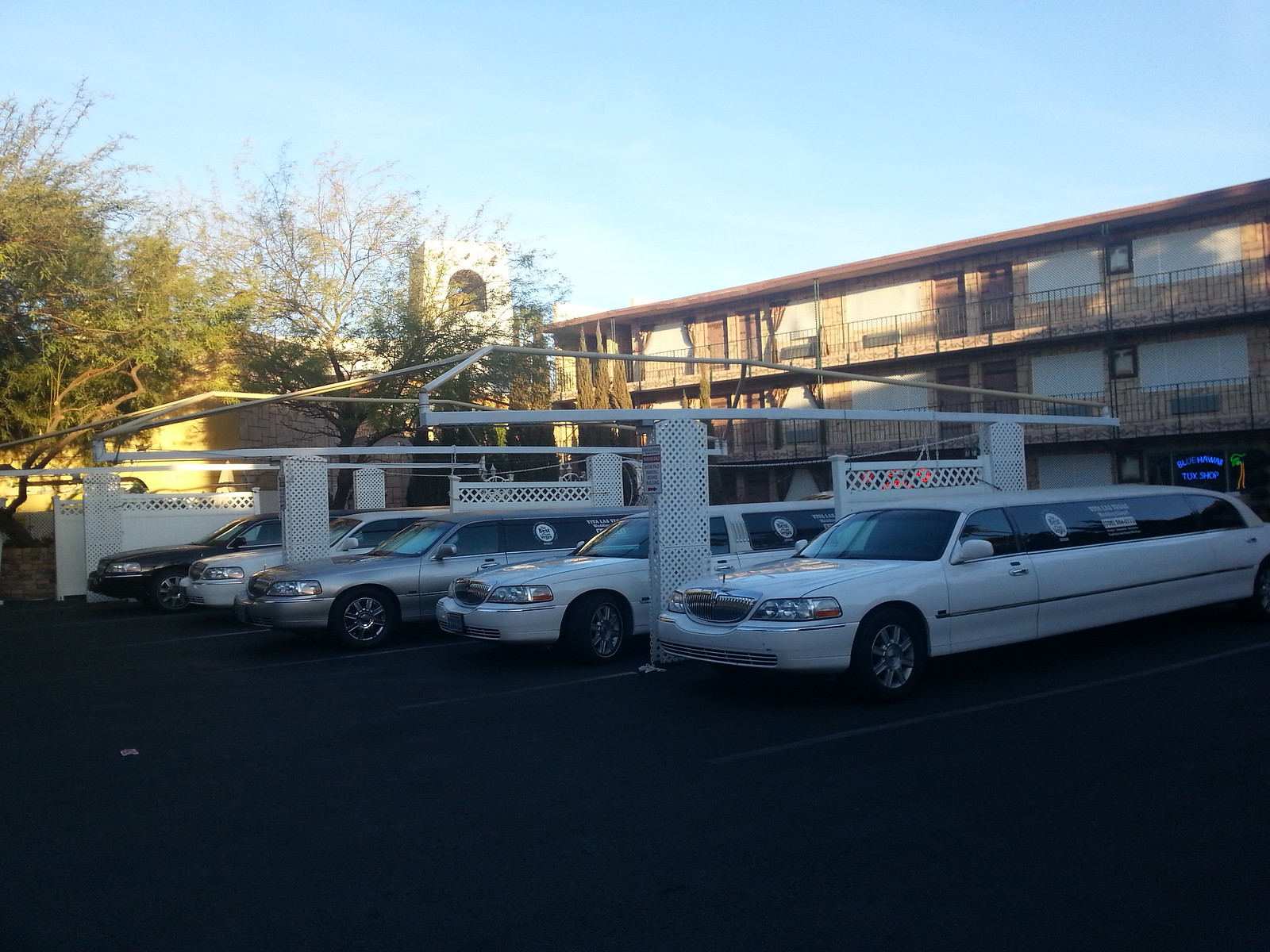This vibrant outdoor photograph captures a clear, blue sky day with a few scattered clouds and trees in the background, framing the scene. Dominating the image is a three-story motel-like structure with outdoor entrances and distinct visible balconies. The building appears aged and sunlit, casting shadows in the foreground. In front of the building, a row of five limousines is lined up in the parking lot. These limousines are in various colors: two are white, one is silver, and one white with the furthest one being black. Each limousine has round logos on the windows and square stickers displayed prominently. White lattice fences and partial fence sections create bay-like structures separating the vehicles. A metal structure, possibly the supports for a roof, is partially visible overhead. To the right side of the photograph, there's a small neon sign that potentially reads "Blue Hawaii Tuck Shop," adding a touch of color to the otherwise serene scenery.